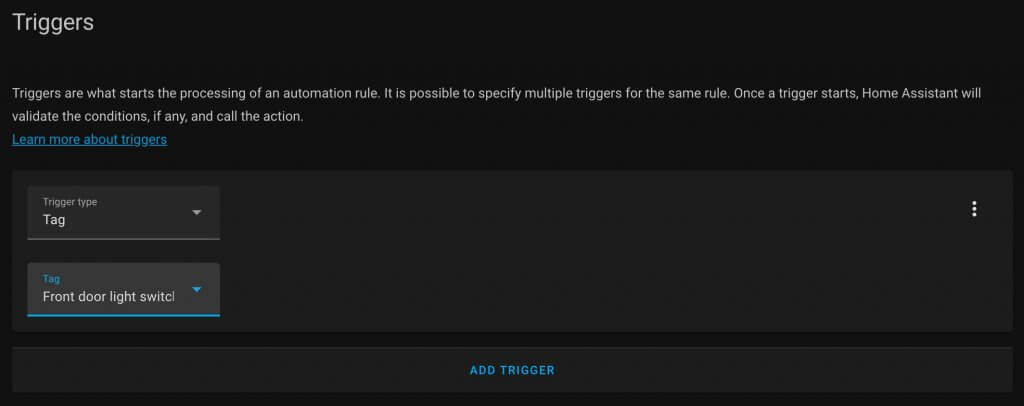### Detailed Caption:

This screen capture displays a configuration interface from what appears to be a home automation software, possibly Home Assistant. The page features a primarily black background with contrasting white text and blue-grey elements for clarity. At the top, a header reads "Triggers," highlighted in bold white text. Below the header, a descriptive paragraph explains that triggers initiate the processing of an automation rule. It mentions that multiple triggers can be specified for a single rule, and once a trigger activates, Home Assistant verifies any conditions before executing the associated action.

A blue hyperlink labelled "Learn more about triggers" provides additional information or resources on the topic. 

Further down, the interface is divided into two main sections:
1. **Trigger Type:** Accompanied by a drop-down menu that enables the selection of different trigger types.
2. **Tag:** This section is highlighted with a blue border and currently set to "Front Door Light Switch," indicating the specific device or event that will activate the rule.

At the bottom of the interface, a clickable blue-text option "Add Trigger" allows the user to add more triggers to the automation rule. The color scheme consists of black, white, blue, and various shades of gray, providing a clean and professional appearance conducive to ease of use and readability in a security configuration context.